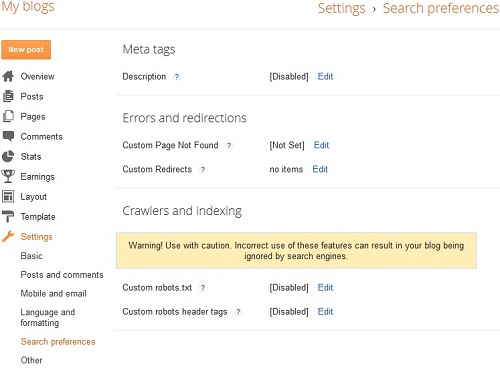The image depicts an intricate layout of a blog management dashboard with a predominantly white background. In the top left corner, the text "My Blogs" is displayed in orange. Directly below this heading is a tab labeled "New Post," featuring white text set against an orange box.

Beneath the "New Post" tab, there is an assortment of navigational options: an overview icon resembling a small house, and links for Posts, Pages, Comments, Stats, and Earnings. The Stats section is highlighted by a pie graph icon. Adjacent to this, there’s a trophy image symbolizing achievements or milestones.

Further down, the layout and template options are presented alongside an orange wrench icon indicating settings. This segment includes links for adjusting basic posts and comments, mobile and email settings, language and formatting preferences, search preferences, and other settings—each accompanied by orange icons for consistency.

Moving to the top center section, the word "Meta Tags" is prominently displayed in larger text. Below it, in smaller lettering, the word "Description" appears with a question mark next to it. To the right, the word "Disabled" is enclosed in parentheses, followed by an "Edit" option in blue. A faint line beneath this section demarcates a new category.

The next category is "Errors and Redirections," which shares the same text size as "Meta Tags." Listed under this are options for managing a Custom Page Not Found, marked with a question mark, and a corresponding "Edit" button in blue. Further down, "Custom Redirects" is noted, with a statement indicating no items and an accompanying "Edit" button.

The bottom section addresses "Crawlers and Indexing," highlighted by a yellow warning box advising caution due to potential consequences on blog visibility by search engines. Within this category, "Custom robots.txt" and "Custom robots header tags" are mentioned, both marked disabled and paired with question marks for additional information.

The entire interface is set against a clean white backdrop, enhancing readability and visual organization.